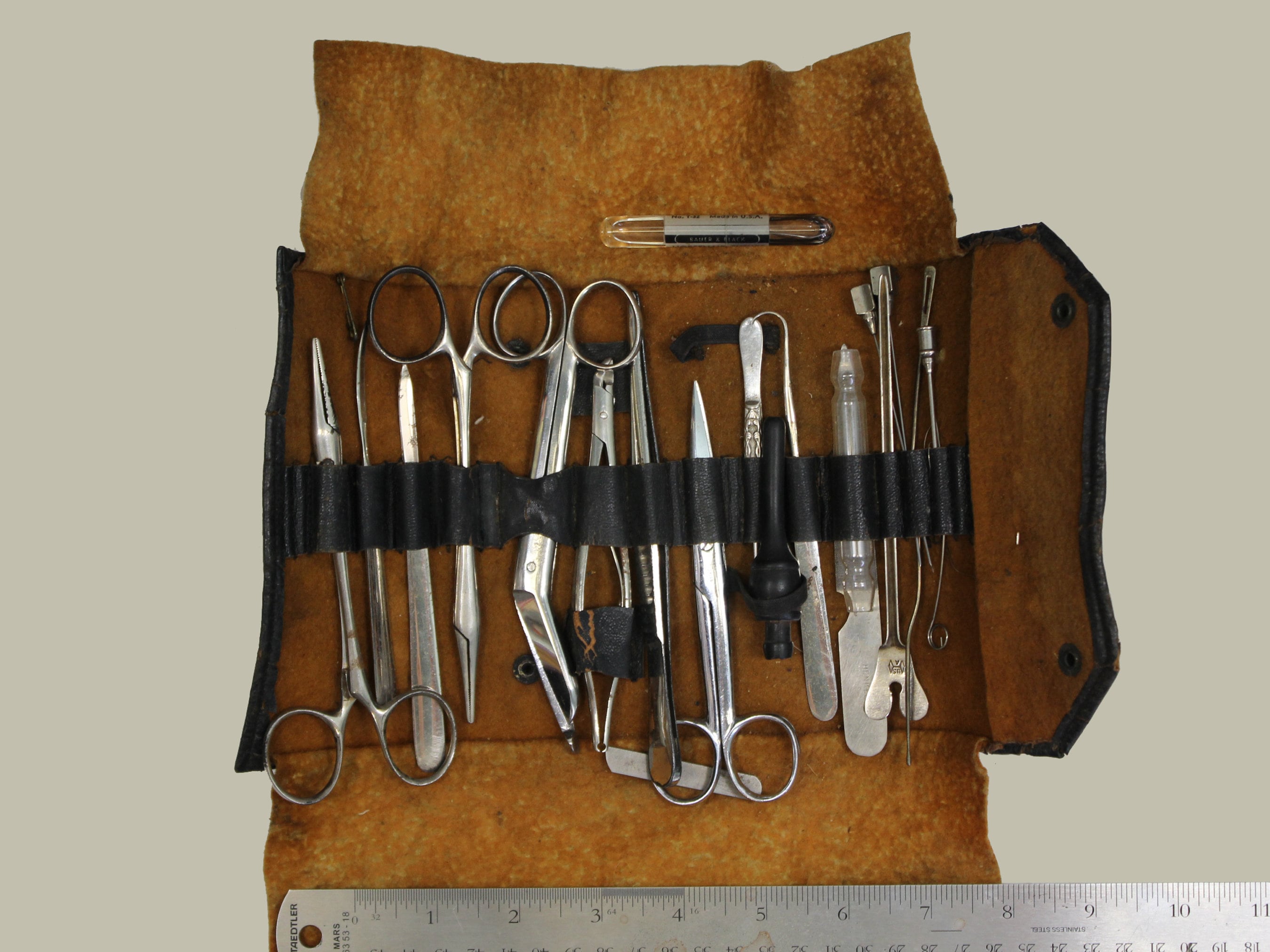The photograph features an old-fashioned, leather-bound medical or dental tool kit, meticulously arranged and displayed. The casing, made of brown leather with a lighter tan interior, reveals a collection of stainless steel instruments when opened. These instruments, held in place by a central black strap, include various types of scissors, tweezers, clamps, blades, picks, and small scoop-shaped spatulas, all reminiscent of barbering or medical tools. The kit has two dark snaps on the right side for secure closure and is lined with black edging. At the bottom of the photograph, a silver metal ruler extends to the right, indicating that the kit measures approximately 8 to 9 inches across. The background of the image is a light beige color, enhancing the vintage and clinical feel of the tool kit.